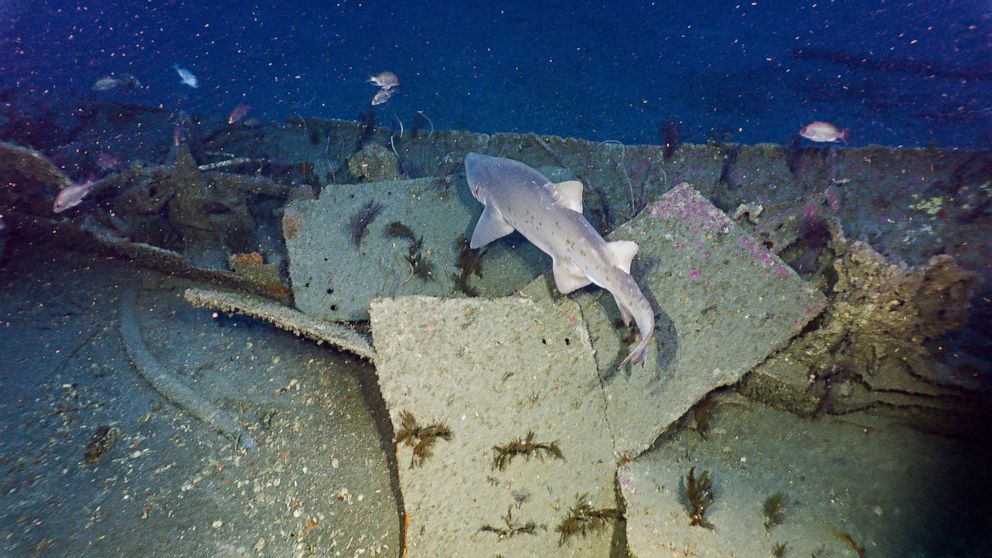This underwater photograph captures a sunken shipwreck lying on the ocean floor, encrusted with sea plants and coral. The sizable wreck, covered in metal fragments and underwater flora, is teeming with various types of fish, vividly highlighted by a diver’s light against the dark blue water. At the center of the scene, a smaller-sized gray shark glides above the wreckage, surrounded by swarms of smaller fish. The wreck has been submerged for quite some time, providing a thriving habitat for diverse marine life.